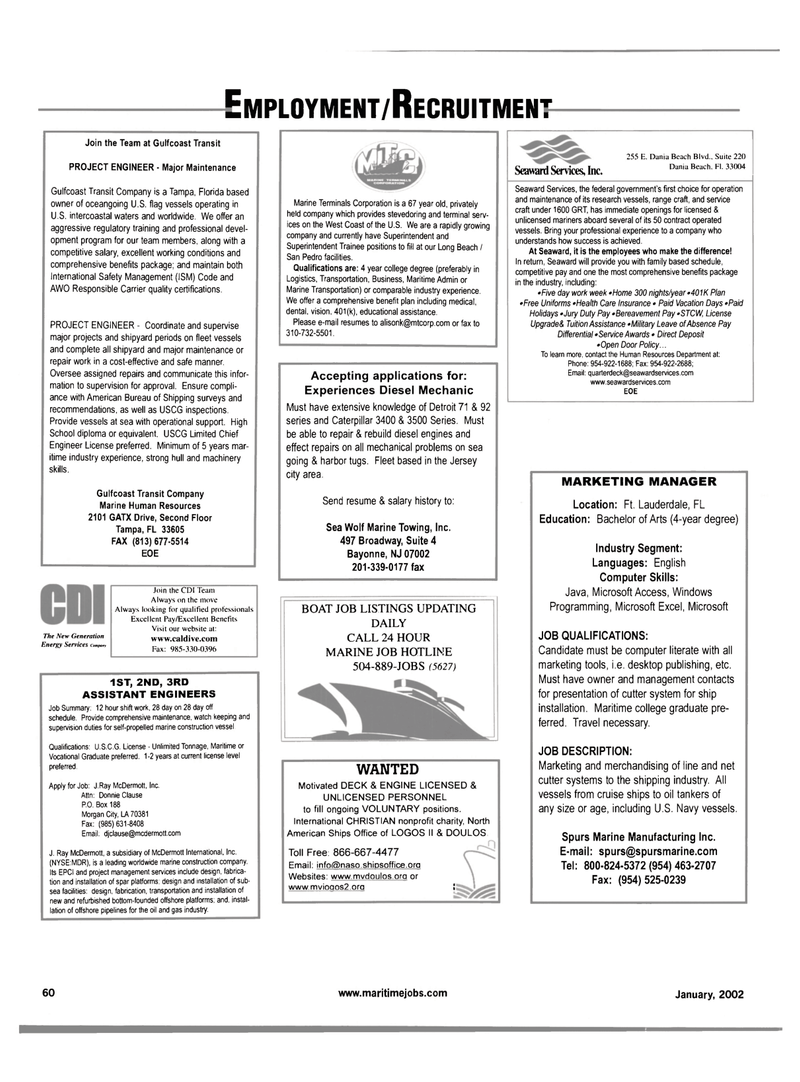The image depicts a page from a pamphlet focused on employment and recruitment, prominently titled "Employment / Recruitment" in bold black text at the top. The page is filled with various advertisements for job opportunities, organized in blocked sections and rectangular boxes. 

The top-left section advertises a position for a Project Engineer in Major Maintenance, with two descriptive paragraphs and an address. Adjacent to this, on the right, are two square-shaped ads of equal height. One of these ads, titled "Accepting Applications for Experienced Diesel Mechanic," includes details about qualifications and job locations. 

Another section on the right promotes C-word Services Incorporated, although the text is partially unreadable. Below this, there's a CDI box listing openings for 1st, 2nd, and 3rd Assistant Engineers. To the right, there are two more boxes: one lists boat job opportunities updated daily with a 24-hour marine job hotline number, and the other seeks a Marketing Manager, detailing the job qualifications, description, address, and contact information.

At the bottom of the page, the date "January 2002" is mentioned alongside the URL "www.maritimejobs.com" and the page number "60." The advertisements collectively offer positions such as Project Engineer, Major Maintenance, Experienced Diesel Mechanic, and various marine-related roles, indicating a strong emphasis on maritime jobs.